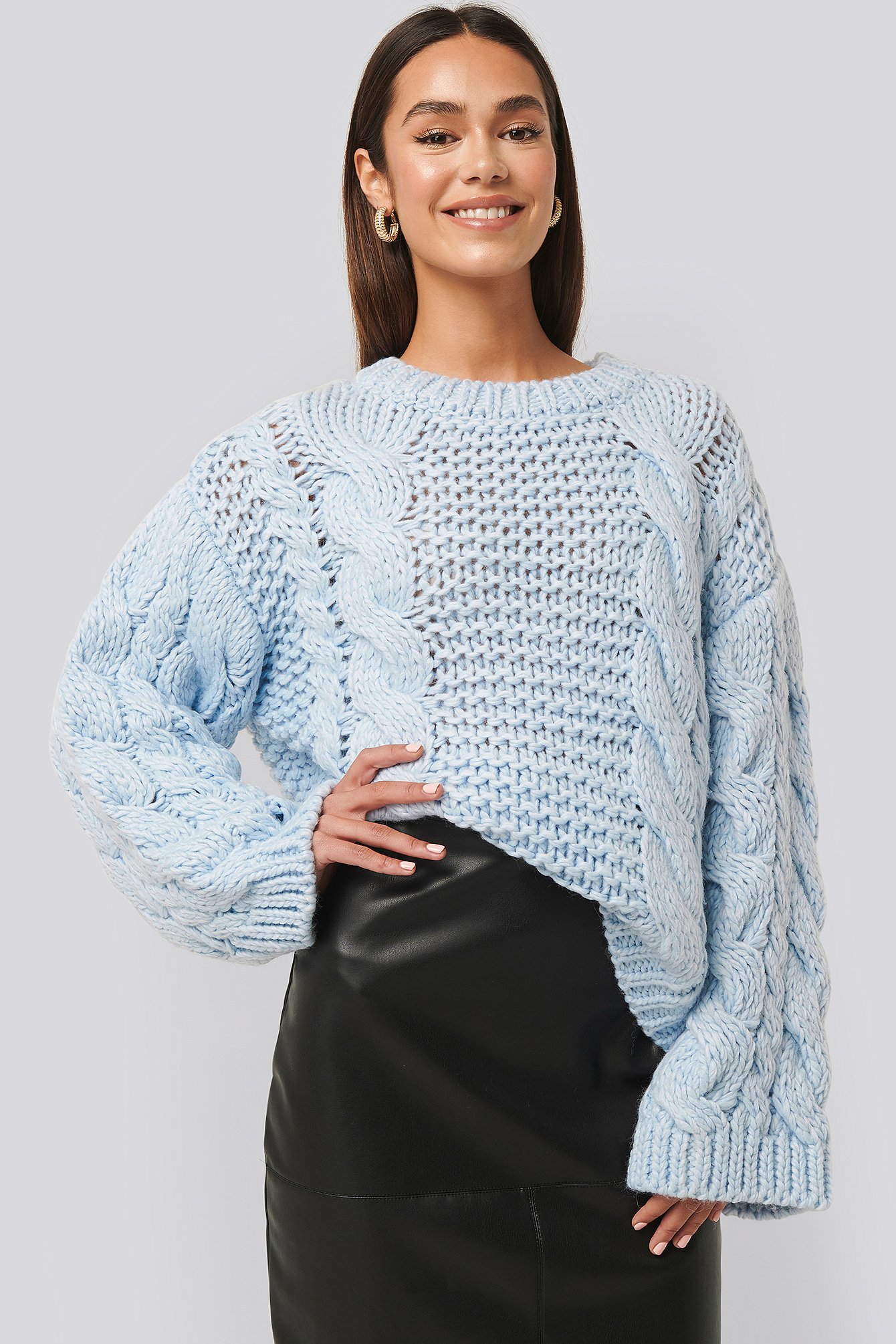This studio photograph captures a young, attractive model in her early 20s, standing confidently against a grey backdrop. She is wearing a highly textured, light baby blue cable knit sweater that looks warm and stylish. Complementing the sweater is a black leather skirt, which is visible from the waist down to mid-thigh. Her right hand rests on her hip, exuding confidence, while her left hand hangs gracefully by her side, showing off her light pale pink manicure. She has long, dark blonde hair, parted in the middle, cascading past her shoulders. Adorned with thick, golden hoop earrings, her look is completed with tasteful makeup and a bright, captivating smile. Her poised and joyful demeanor suggests she is enjoying the modeling session.